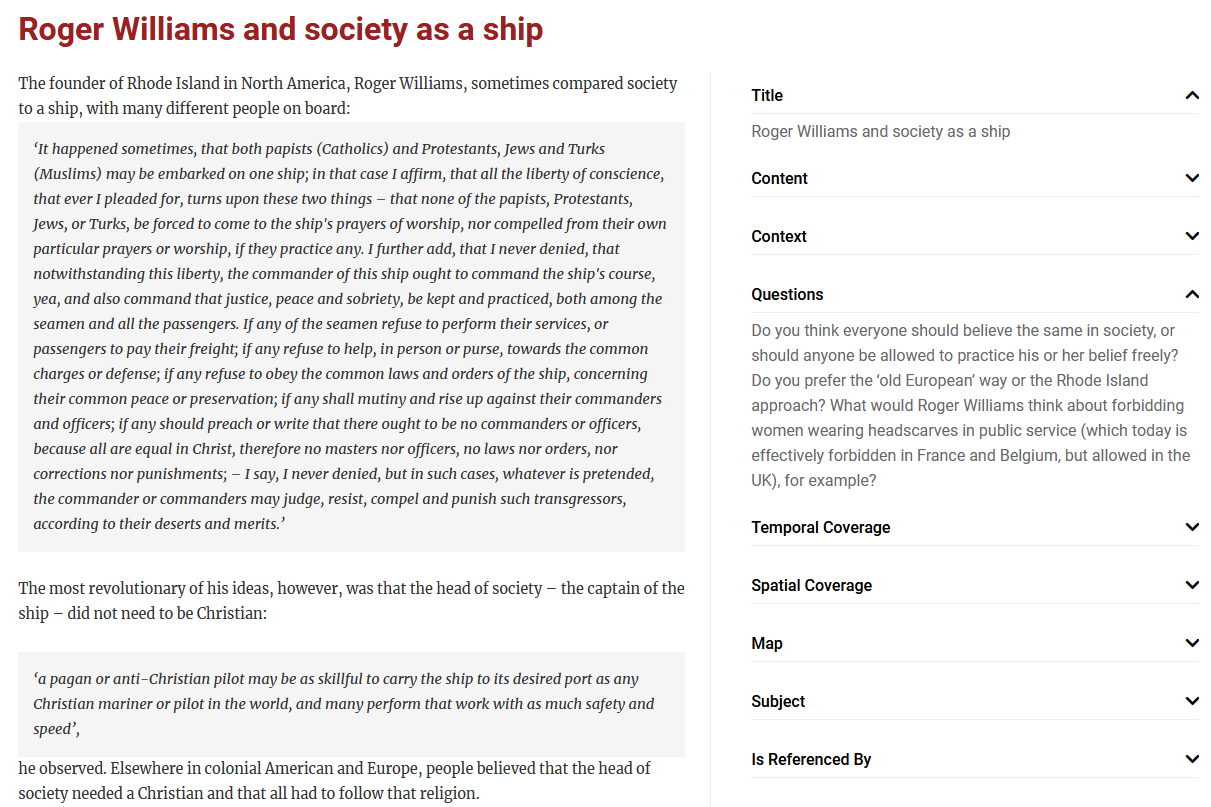The image showcases a detailed screenshot of an article with a layout divided into two distinct sections. On the left side, the main article is prominently featured, adorned with a burgundy title reading, "Roger Williams and Society as a Ship." Below the title, a brief summary in black text introduces Roger Williams, the founder of Rhode Island, who is noted for comparing society to a diverse crew aboard a ship.

Underneath this summary, a substantial, gray-highlighted quote from Williams' writings is prominently displayed. The excerpt begins: "It happens sometimes that both the Papists, that is Catholics, and Protestants, Jews and Turks, that is Muslims, may be embarked on one ship. In that case, I affirm that all the liberty of conscience that I ever pleaded for turns upon these two things, that none of the Papists, Protestants, Jews or Turks be forced to come to the ship's prayers of worship, nor compelled from their own particular prayers of worship." This quote underscores Williams' advocacy for freedom of worship and is accompanied by commentary and additional quotes providing context and supporting his views.

On the right side of the image, various interactive elements are neatly arranged, including the article's title repeated, navigation buttons labeled "Content" and "Context," and sections titled "Questions You Might Ask About It," "Temporal Coverage," "Spiritual Coverage," "Map," "Subject," and "Referenced By." These elements suggest an in-depth and layered analysis of Williams' metaphor and its implications. The screenshot, evidently from an online discussion platform, represents a rare and insightful topic of discourse, emphasizing the enduring relevance of Roger Williams' thoughts on religious freedom and societal diversity.